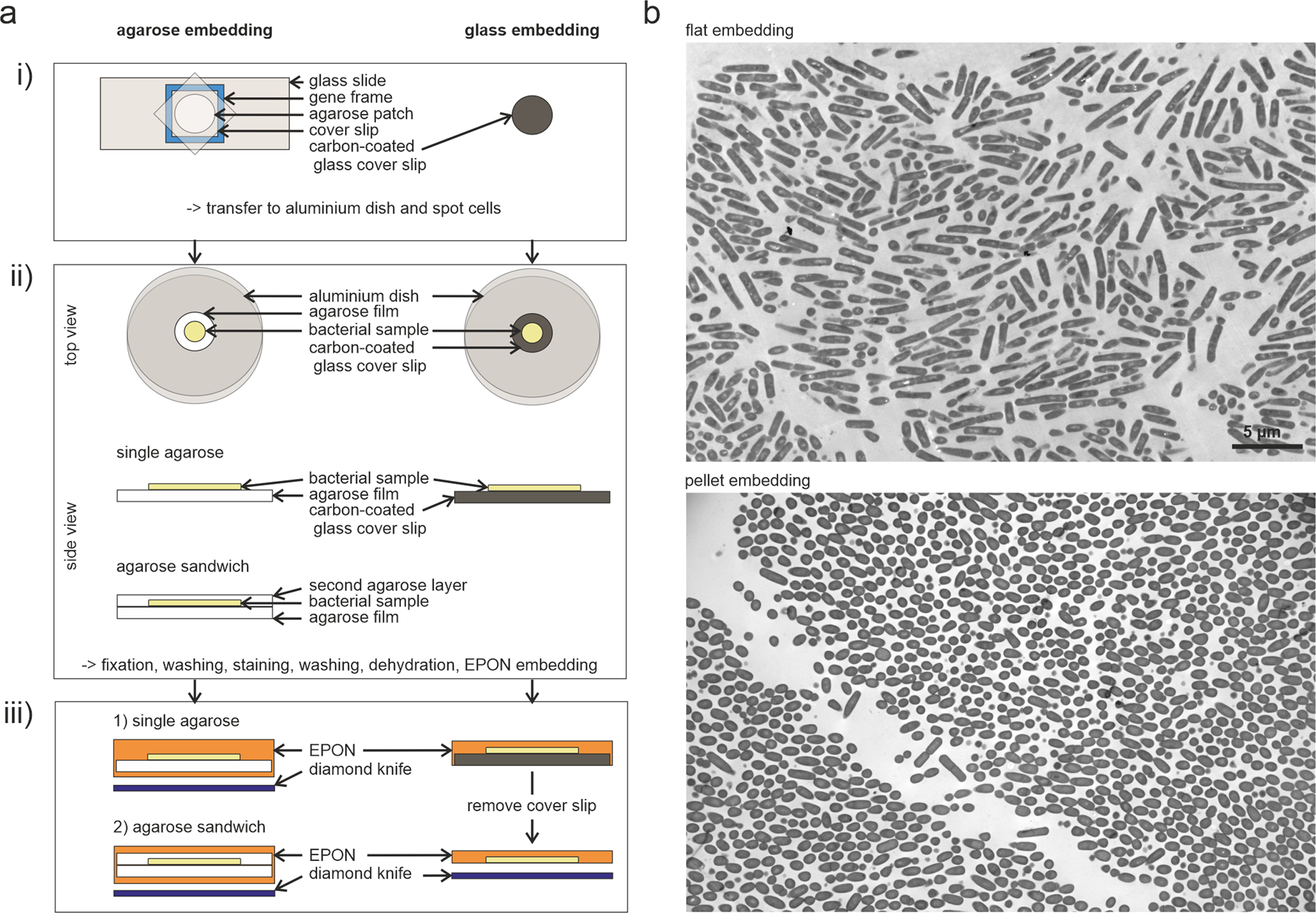This image, appearing as a scientific diagram from a textbook, illustrates methods for embedding samples in transmission electron microscopy to possibly reveal mechanisms of tetracycline. The diagram is divided into two main sections, with methodologies on the left and visualization results on the right.

**Left Side: Methodologies (Section A)**
- **Embedding Techniques:** Two main techniques—`Agarose Embedding` and `Glass Embedding`—are displayed.
    1. **Agarose Embedding :** Depicts a sequence starting with components like a glass slide, a gene frame, an agarose patch, a cover slip, and a carbon-coated glass cover slip. The process description includes transferring to an aluminum dish and spotting cells.
        - **Stage 2:** Shows a top view illustrating components such as an agarose film, bacterial samples, carbon-coated glass cover slip, forming either a "single agarose" setup or an "agarose sandwich."
        - **Stage 3:** Details the embedding stages, including fixation, washing, staining, dehydration, and Epon embedding, with instructions on using a diamond knife to remove cover slips and handle samples.
    2. **Glass Embedding:**
    - Exhibits its specific steps and mentions components like carbon-coated cover slips to highlight sample preparation differences.

**Right Side: Visualization (Section B)**
- **Microscope Readouts:** This section displays the results seen under a microscope.
    - **Top Image: Flat Embedding**
        - Shows a flat embedded sample presenting worm-like structures in darker gray shades against a gray background.
    - **Bottom Image: Pellet Embedding**
        - Displays pellet-embedded samples appearing as jelly bean-shaped darker gray pieces.

This comprehensive diagram underscores the detailed process of preparing and viewing microscopic samples, encompassing embedding methodologies and their corresponding visual results under a microscope.